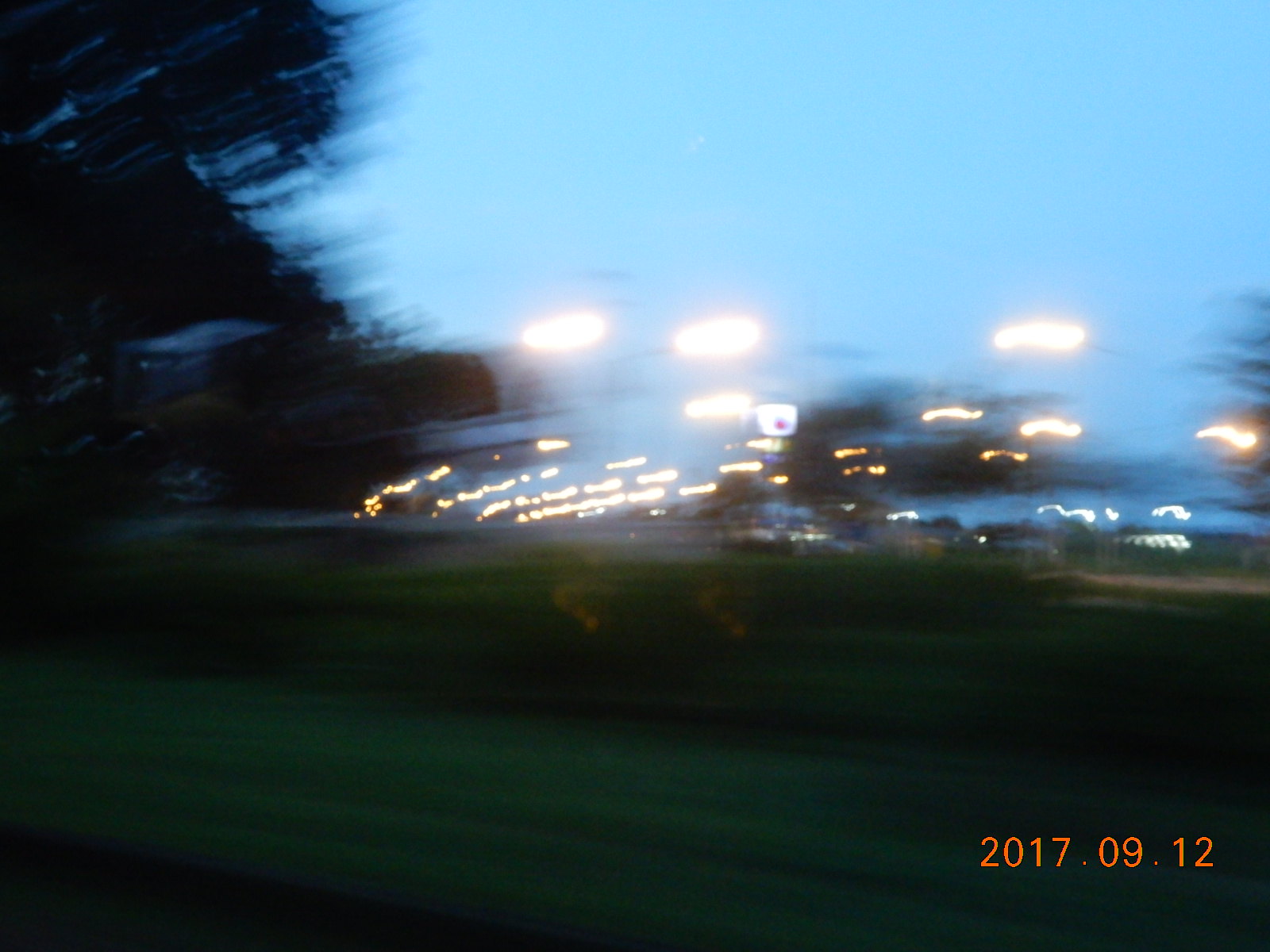A landscape photograph captured during twilight from a moving vehicle, resulting in a blurred effect. The image showcases the indistinct outline of a tree against a backdrop of green grass. In the distance, a clear blue sky transitions into the early evening, dotted with the scattered, glowing lights of a city or a series of street lamps. A timestamp at the bottom of the photograph reads "2017-09-12," marking the date of this fleeting moment.